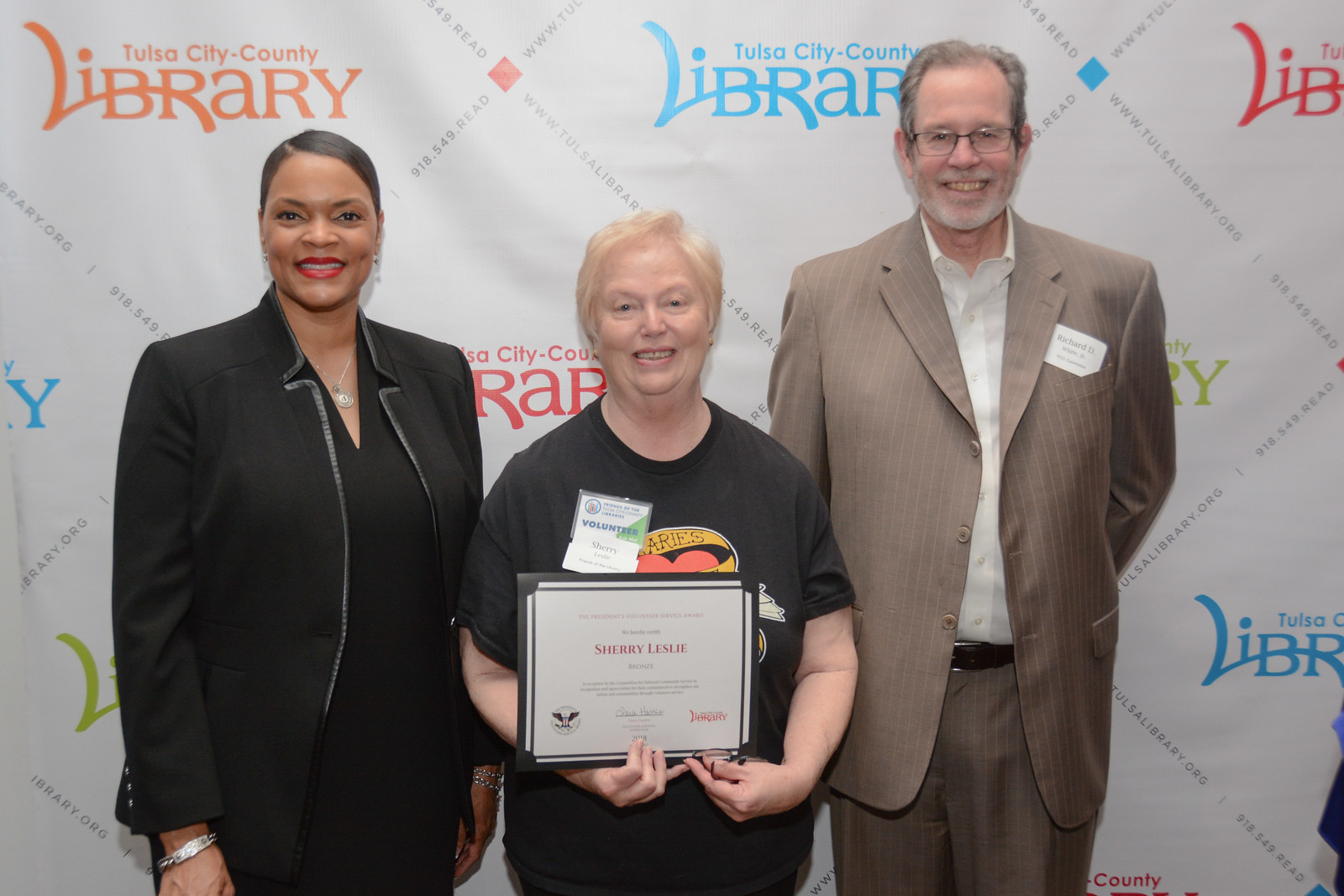The image depicts three smiling individuals standing in front of a white backdrop covered with the words "Tulsa City County Library" in various colors such as orange, blue, and red. The backdrop also features the library's contact information, including the website "www.tulsalibrary.org" and phone number "918-549-READ," repeated in a diamond pattern. In the center stands an elderly woman with short blonde hair, wearing a short-sleeved black shirt. She holds a certificate with her name, "Sherry Leslie," and sports a name tag labeled "volunteer." She smiles warmly at the camera. On her left is a taller, middle-aged black woman dressed in a black business suit, also smiling. To the right stands an older white man with gray hair and glasses, dressed in a tan suit without a tie and a white dress shirt. The typography of the word "Library" in the backdrop features a unique design where the bottom part of the "L" extends under the "I," passes through the center of the "B," and ends at the rounded part of the "R."